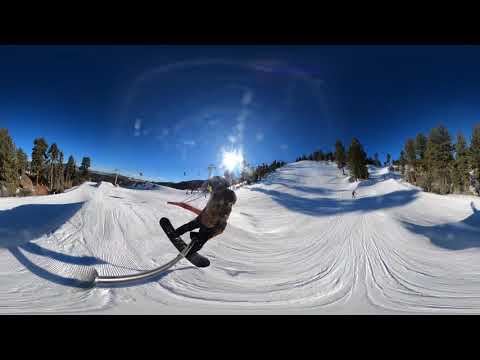This color photograph, bordered by black frames at the top and bottom, vividly captures a dynamic scene of snowboarding on a picturesque winter day. In the foreground, a snowboarder, adorned in a snowsuit with a black snowboard, executes a maneuver with the front end of their board lifted into the air. The pristine white snow beneath them shows the well-trodden paths of previous adventurers, and trees exhibiting vibrant green hues line the path down the hill, reflecting off the snow.

Adjacent to the snowboarding action, a skier can be seen navigating the trail, adding to the lively atmosphere. The brilliance of the scene is accentuated by the sun, which shines brightly, creating a sun glare directly above the snowboarder and illuminating the vivid blue sky that holds no clouds. In the distance, a snow-covered mountain stands majestically, accompanied by a ski lift with two towers and two cars traversing the cable, highlighting the bustling activity of the area. The photograph also interestingly distorts space slightly, giving a unique, curved perspective to the landscape, and while it is unsigned and undated, it encapsulates the serene yet exhilarating essence of winter sports in a mountainous terrain.